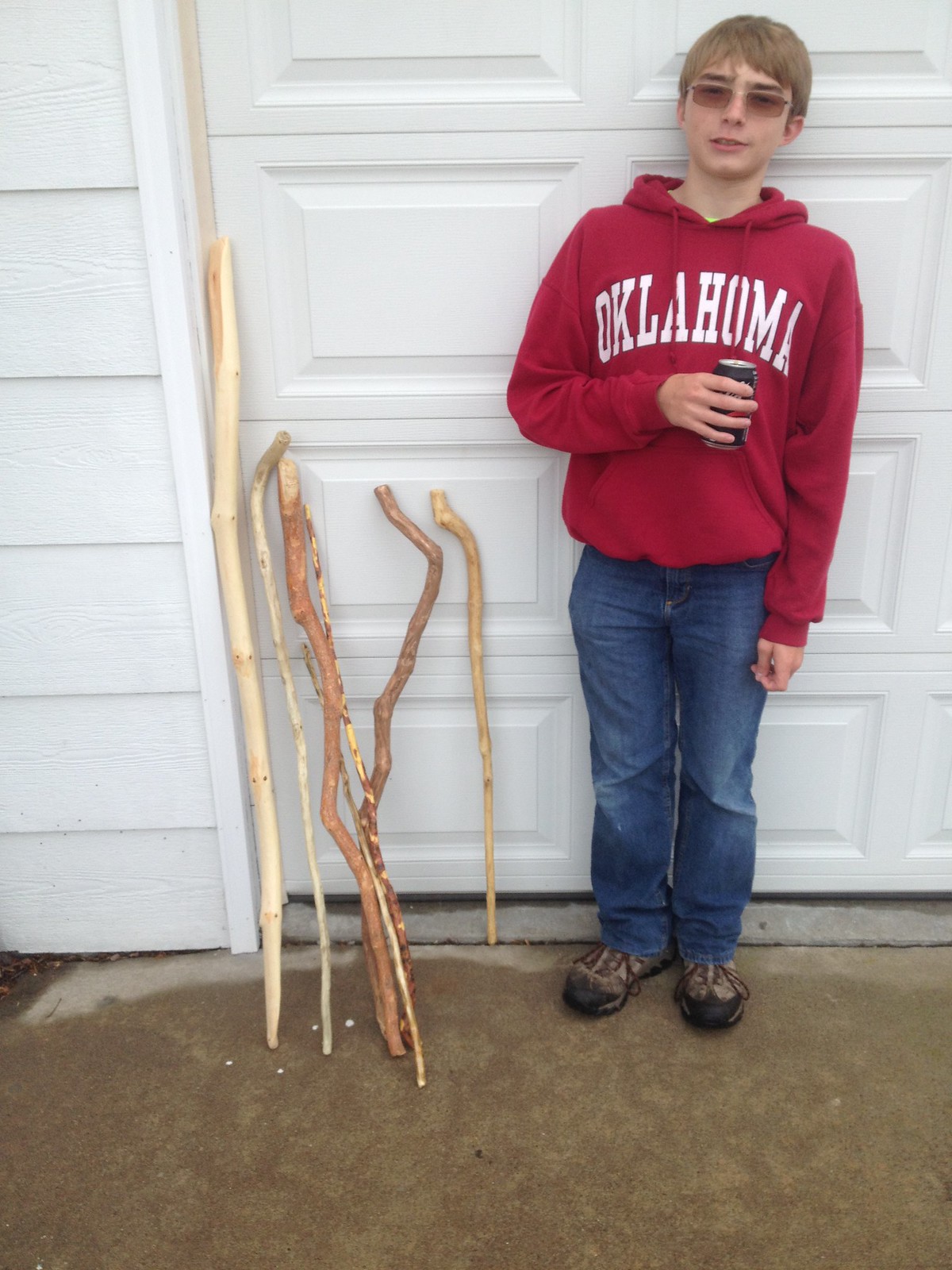The image is a color photograph in portrait orientation, showcasing a young man, roughly 13 or 14 years old, standing firmly in front of a white garage door characterized by its grid-like pattern of recessed panels. The setting includes horizontal siding to the left of the garage door, part of the house or property. The boy has light brown to dirty blonde hair, which is cut short to his head, and he wears a pair of semi-transparent sunglasses. Draped in a red hooded sweatshirt with white pull cords hanging down the front, the sweatshirt prominently features the word "OKLAHOMA" in white, arching across the chest area. He pairs this with dark blue jeans that exhibit some fading around the knees and brown walking shoes. In his left hand, he holds a can, possibly soda. To his right, a collection of variously colored and types of walking sticks, including light brown, dark brown, and a taller, cleaner walking staff, lean against the garage door, suggesting they might be homemade from found wood.